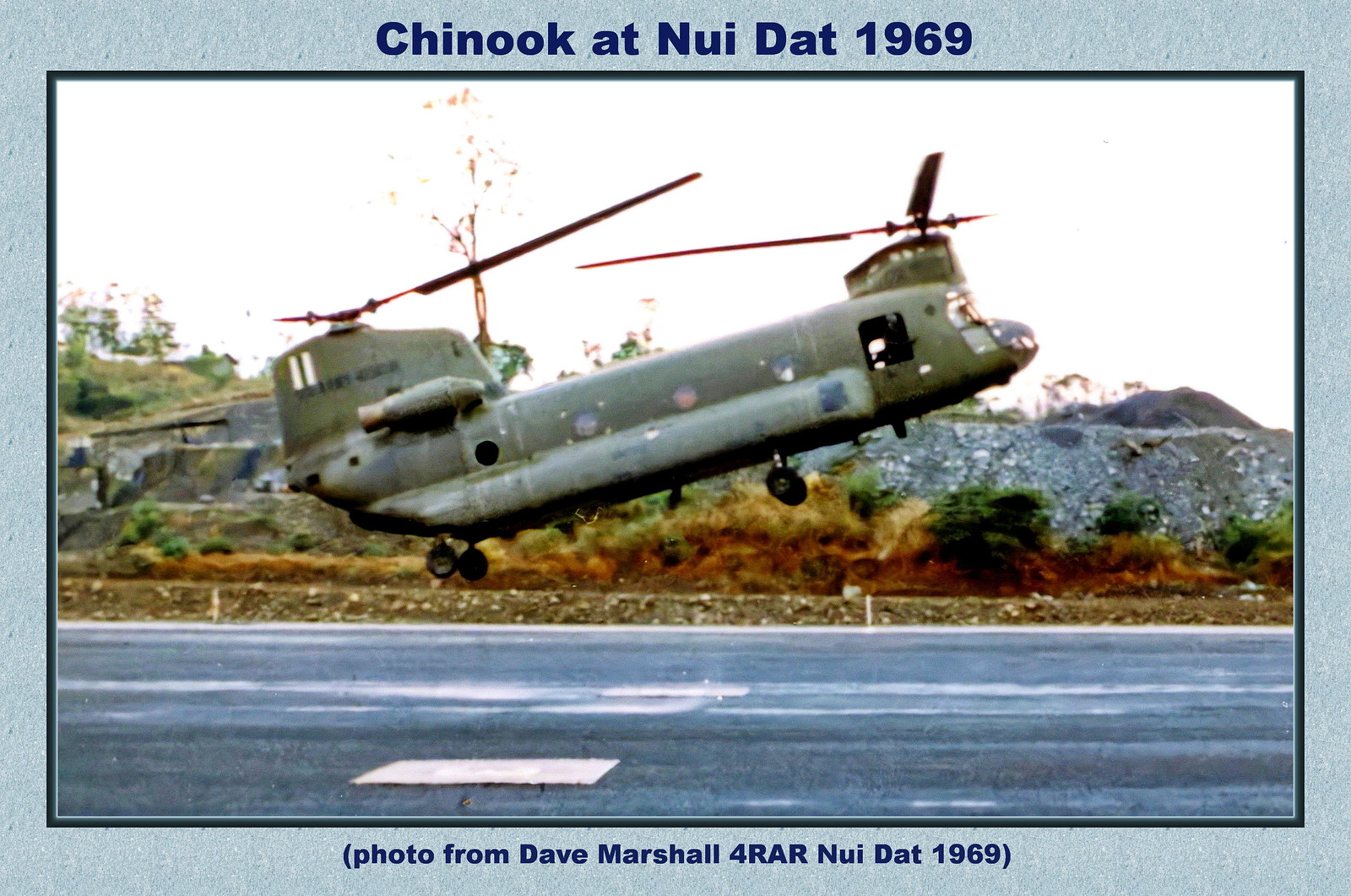The image appears to be an aged photograph surrounded by a blue, sandy-textured border. At the top of the border is an inscription in navy blue font that reads "Chinook at Nui Dat 1969." At the bottom, it says "Photo from Dave Marshall for RAR Nui Dat 1969." The scene depicts a green military-style Chinook helicopter, identifiable by its black propellers, either taking off or landing just above a gray and black asphalt landing strip. This historical image, likely from the Vietnam War era, shows the helicopter in a stationary position against a backdrop of trees, rocky hills, bushes, and small gravel piles, adding to the vintage ambiance of the photograph.